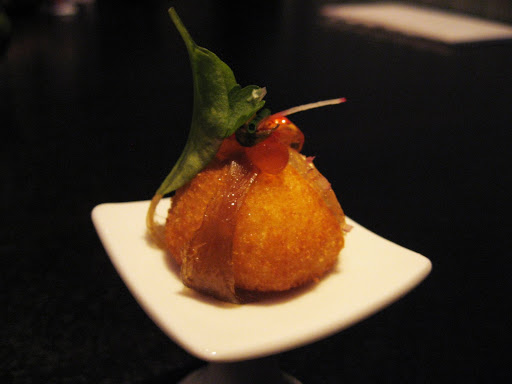The image features a close-up of a single gourmet pastry or food item placed on a small white, diamond-shaped porcelain plate. The pastry is round and golden brown with a shiny exterior, suggesting it may be coated in sauce or butter. At the top center of the pastry, there are three semi-translucent red circular shapes, possibly berries, adding a pop of color. A vibrant green leaf, likely mint, extends from the back, contrasting against the warm tones of the pastry. The plate rests on a sleek, black shiny tabletop with hints of white and gray in the blurred background, possibly indicating a placemat and seating area. The whole setup exudes an elegant and refined presentation, emphasizing the delicacy and gourmet nature of the dish.